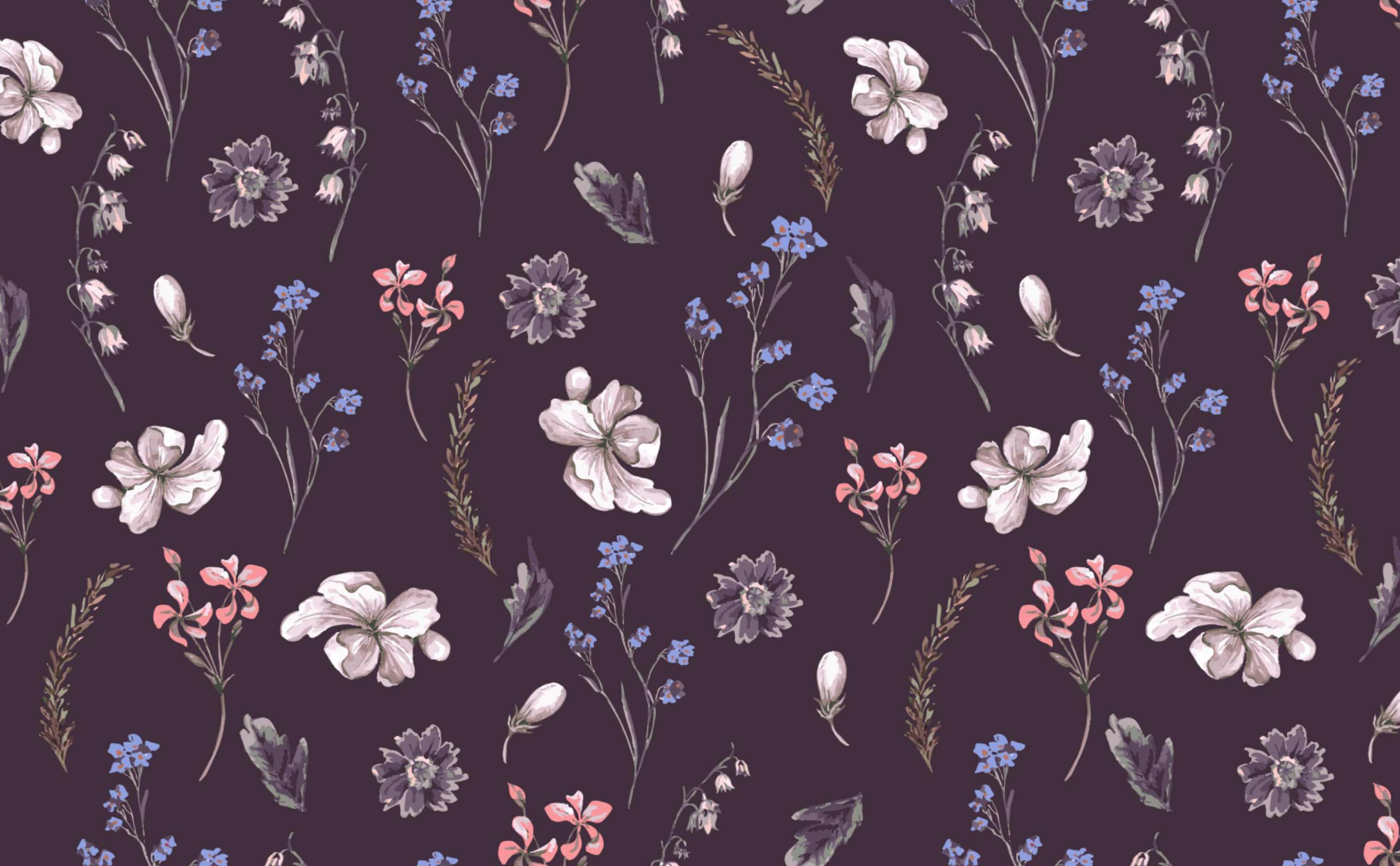The image displays a detailed and intricate wallpaper design with a dark gray-black background. Scattered across the background are various types of plants and flowers, repeating in a somewhat irregular but aesthetically pleasing pattern. Dominating the scene is a white flower with five petals, lacking stems or leaves. Adding vibrant touches to the composition, there are small green-stemmed plants with delicate blue flowers and similar plants bearing tiny pink flowers. Among these, a unique, purple-petaled flower catches the eye. The design also includes dark grayish flowers and small, very fine leaves sprouting from stems. Adding further texture, white bulbous shapes appear sporadically, resembling unbloomed flowers, and a much darker gray leaf, distinct with a feathery shape, is interspersed throughout. The combination of these elements creates a complex and lively pattern that balances both light and dark tones, making the wallpaper rich and visually engaging.